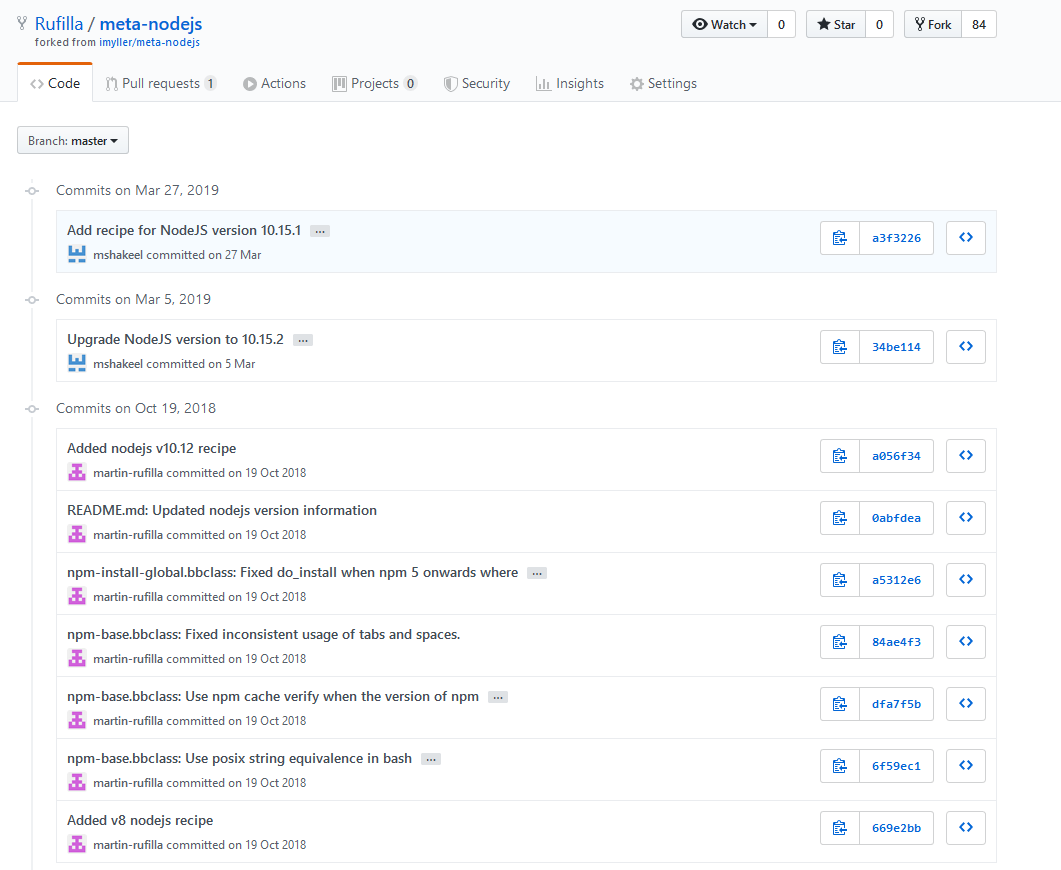Here is a cleaned-up and detailed caption based on the provided voice description:

---
Screenshot of the Rufilla website interface.

In the upper left-hand corner, the "Rufilla" logo is prominently displayed. Below the logo is a breadcrumb navigation path in blue font, reading "Rufilla / meta-node-gs." Underneath the breadcrumb, the path continues with "fort / from" and then "iMillerMeta / noedgs."

Directly below this navigation are several tabs for different sections of the project: "Code," "Pull Requests," "Actions," "Projects," "Security," "Insights," and "Settings." The "Code" tab is currently selected, indicating the viewer is on the code page.

On the left, beneath the tabs, a dropdown menu labeled "Branch: master" is visible, allowing users to switch between different branches of the repository. Below this dropdown, a list of commits is displayed.

The first item in the commit list is dated March 27, 2019, with the comment "Add Recipe for Node.js Version 10.51." The following item in the list is dated March 5, 2019.

The interface is clean and structured, allowing for efficient navigation and management of the repository.

---